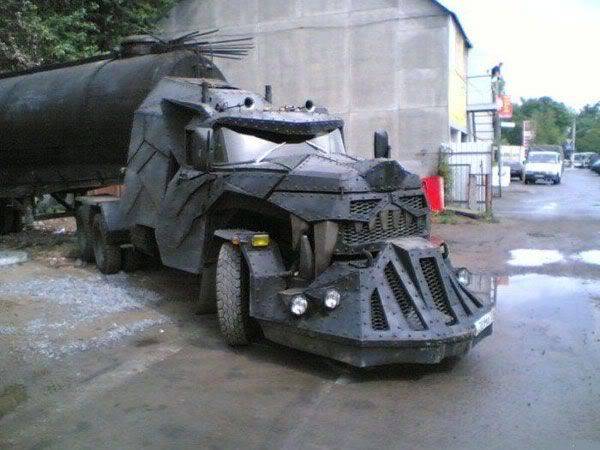The image showcases a heavily armored tanker truck, likely reminiscent of a vehicle from an action movie set. The truck, a multi-wheeled semi-trailer type, is enveloped in gray plates of armor and has an imposing front grille designed to resemble a battering ram. The battering ram is sloped at the bottom for pushing obstacles and features a menacing, tooth-like effect. The vehicle's cab features two prominent horns on top, dual windshield wipers, and numerous smaller-than-average tires. It hauls a large, black cylindrical container, possibly for oil or gasoline. The truck is parked on a dirt surface beside a gray concrete building, likely part of a construction site or factory. Above the truck, leaves from a nearby tree are visible. In the background, there’s more industrial scenery, including additional vehicles and a staircase with a person leaning over the railing. The overall setting appears rugged, reinforcing the vehicle’s formidable design.